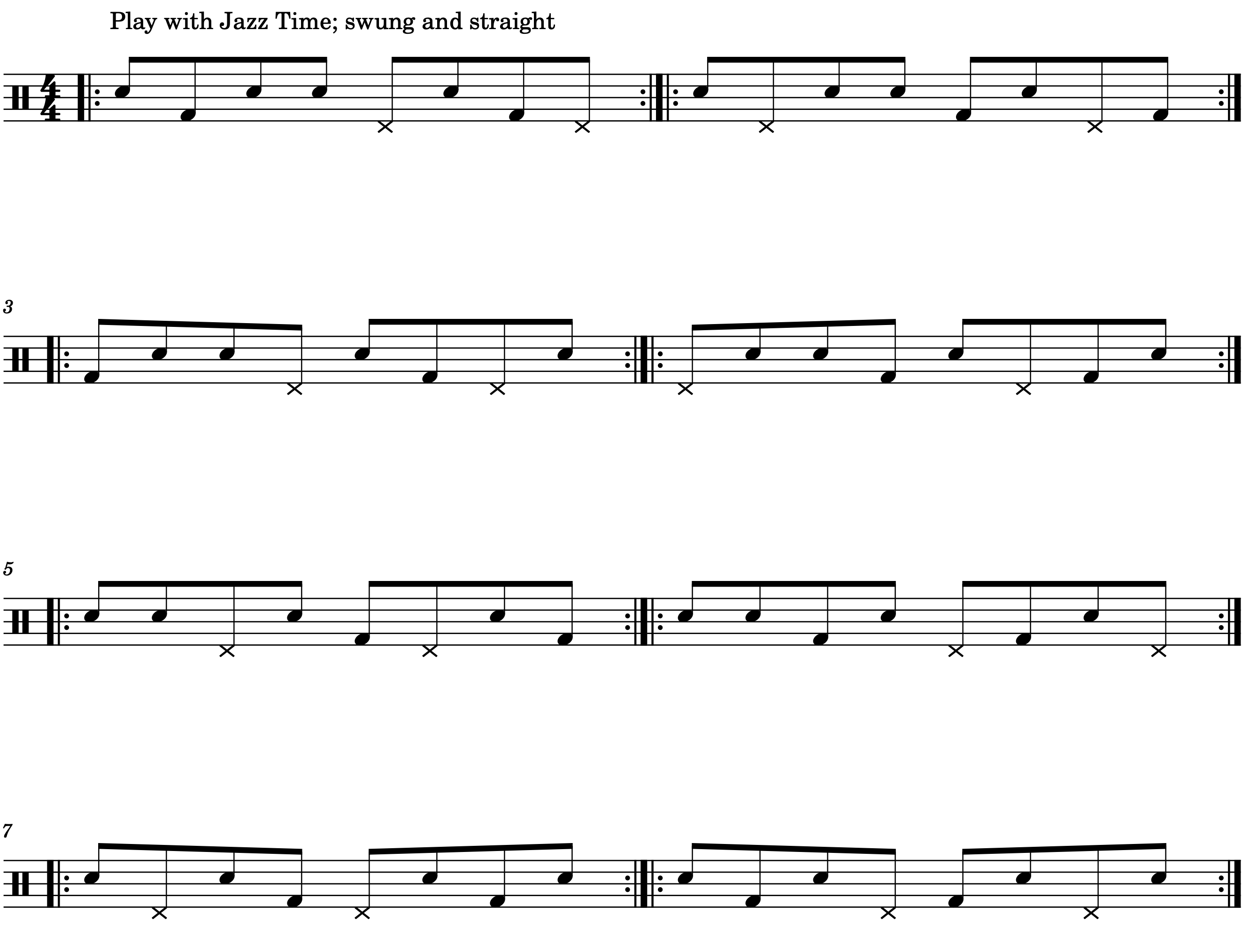The image depicts a simple, black-and-white sheet of music, commonly found in a music book or beginner's class. The sheet consists of four rows, each corresponding to a bar of music. At the top of the sheet, in small black text, it reads, "Play with Jaztime; swung and straight." 

The first row indicates a 4-4 time signature and contains four quarter notes, represented as black dots at the ends of vertical lines, connected to a horizontal bar. Each of the four bars is structured with five horizontal lines resembling guitar strings, upon which the musical notes are placed. 

The subsequent rows are labeled with the numbers 3, 5, and 7, respectively, and each contains its own set of musical notes. The layout showcases the sequencing of different time signatures and rhythms, essential for understanding musical timing and phrasing in jazz music.